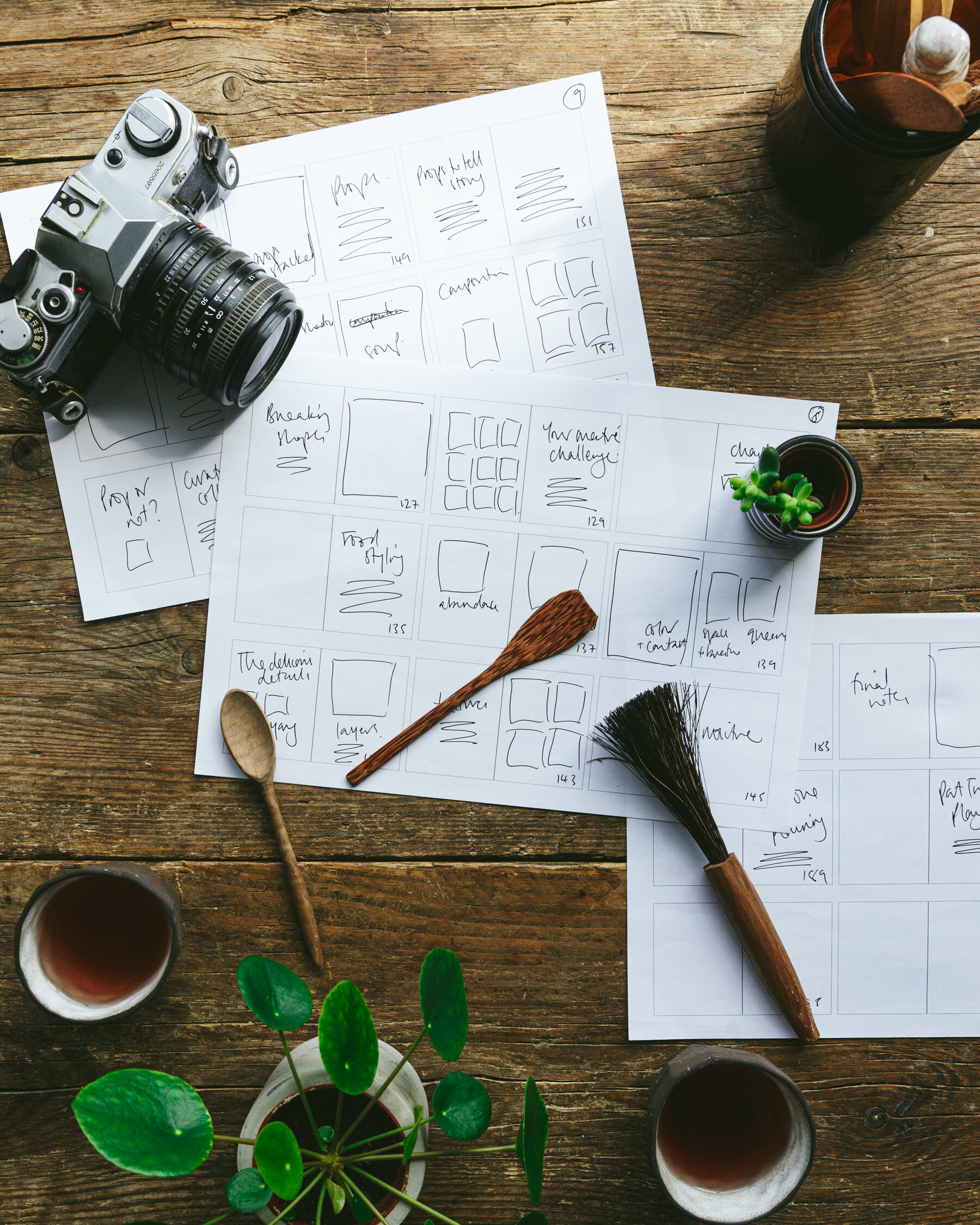In this captivating image, captured in portrait orientation from a top-down perspective, three overlapping pieces of white paper sit on a dark brown rustic wooden table. The papers are divided into grids, each illustrating different methods of drawing squares. Intricate details are evident, though the annotations within the boxes are illegible. 

On the upper left of the image lies an old-school camera with a long black lens, reminiscent of film cameras from a bygone era. On the upper right, atop one of the papers, rests a can housing a green plant with circular leaves. Adjacent to the plant are two wooden spoons, one with a flat edge and the other with a rounded edge, as well as a brush with a wooden handle and black bristles.

Towards the center, a succulent in a dark container adds a touch of greenery. At the bottom of the image, on either side, two cups with an amber-colored liquid suggest tea, nestled in brown containers with white interiors. Centrally placed, a pot with a yellow exterior and green, round-leaved plant further complements the serene, creative setting. The entire scene unfolds atop a richly textured wooden platform, evoking a sense of warmth and artistry.